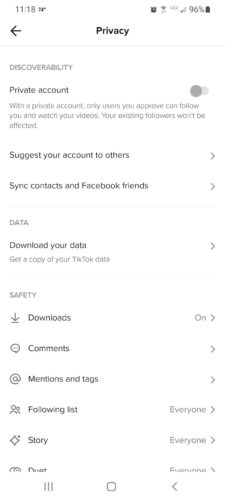This screenshot from a cell phone, though slightly blurry, depicts a settings page against a white background with black text. In the upper left corner, "1118" denotes the time. In the upper right corner, icons display that the battery level is at 96% and the signal reception shows one bar.

The page is titled "Privacy" in bold black text, positioned just below the top row of icons, with an arrow pointing left beside it. Underneath this heading, "Discoverability" is listed in light gray text, followed by the status "Private Account," with a toggle button currently set to the left. There's an explanatory note indicating that with a private account, only users who are approved can follow and view the user's videos, with existing followers remaining unaffected.

Further down, various settings options are available: "Suggest your account to others," "Sync contacts and Facebook friends," and "Data." The "Data" section includes an option: "Download your data" to get a copy of your TikTok data.

The "Safety" section lists several settings: "Downloads are on," "Comments," "Mentions and tags," "Following list," with all settings allowing "Everyone" to interact. Similarly, the "Story" setting is also configured to "Everyone."